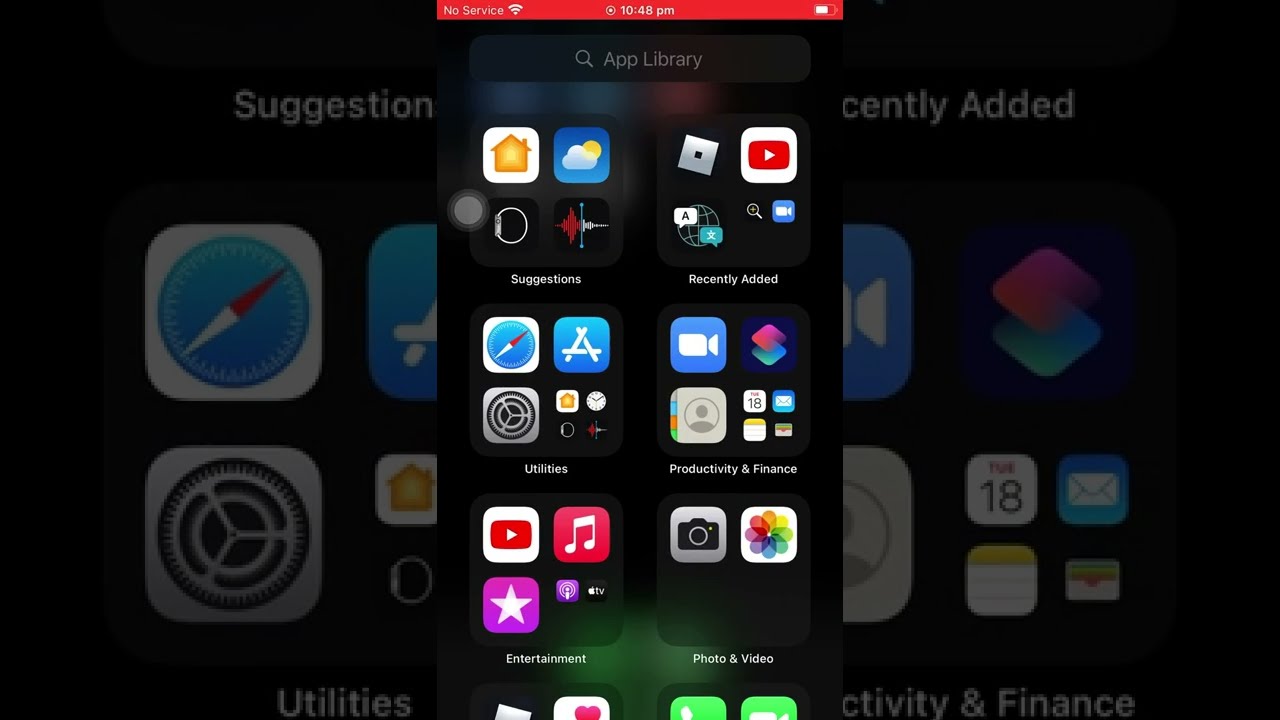The image is a detailed screenshot of an iPhone screen, prominently featuring the "App Library" interface. The background is a black screen displaying various app icons organized into two horizontal rows. At the top, partially obscured text suggests the categories "Suggestions" and "Recently Added." Beneath these, other categories such as "Utilities," "Productivity and Finance," and possibly more are visible, though some text is blocked by a virtual cell phone screen overlay.

The overlay itself is the clearest part of the image, displaying a simulated cell phone screen with the "App Library" header at the top. Below this header, six distinct boxes, each containing grouped app icons, can be seen, although the text labels beneath the icons are small and hard to read. The categories in these boxes include "Suggestions," "Recently Added," "Utilities," "Productivity & Finance," "Entertainment," and "Photo & Video." The screen also shows typical iPhone status elements like the time (10 PM) and "No Service" indicator, along with a red top bar indicating either screen recording or mobile hotspot usage. The bottom part of the virtual cell phone screen is cut off, suggesting there might be additional boxes with app icons that are not fully visible. The image is rich in colors, featuring shades of black, red, silver, gray, blue, orange, purple, lime green, and pink, contributing to its detailed visual presentation.